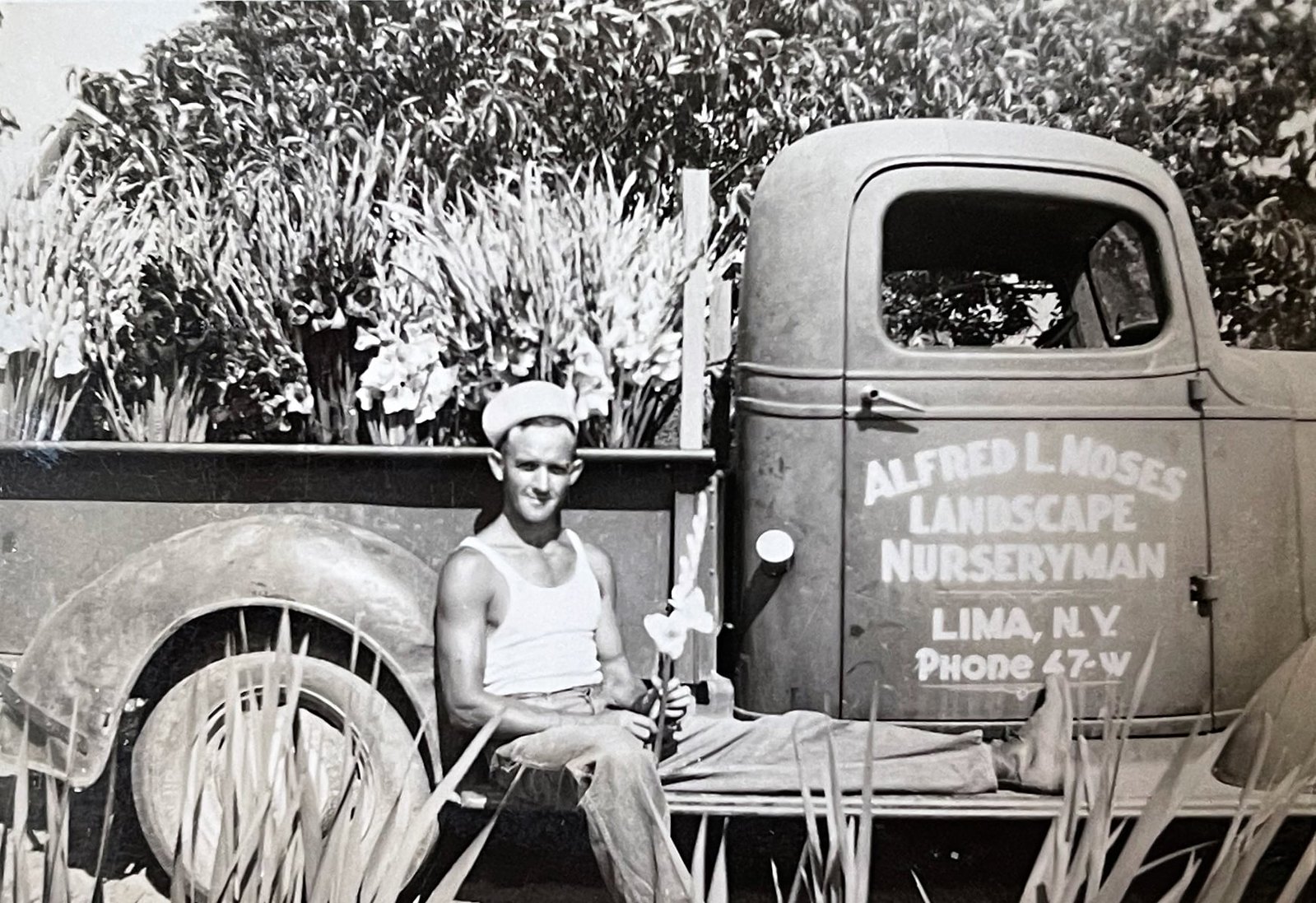A historical black and white photograph captures a man posing in front of a vintage truck, which appears to be promoting his landscaping and nursery business. The man, potentially Alfred L. Moses, is likely the proprietor of the business, as indicated by the large advertisement emblazoned on the truck's side. The ad reads, "Alfred L. Moses, Landscape Nursery Man, Lima, New York," complete with the contact phone number "47W." The backdrop comprises a verdant array of overgrown trees and various plants, emphasizing the connection to his nursery business. The scene is bathed in an aura of antiquity, further highlighted by the aged appearance of both the truck and the photograph. This image serves as a nostalgic glimpse into early 20th-century American entrepreneurship and advertising.